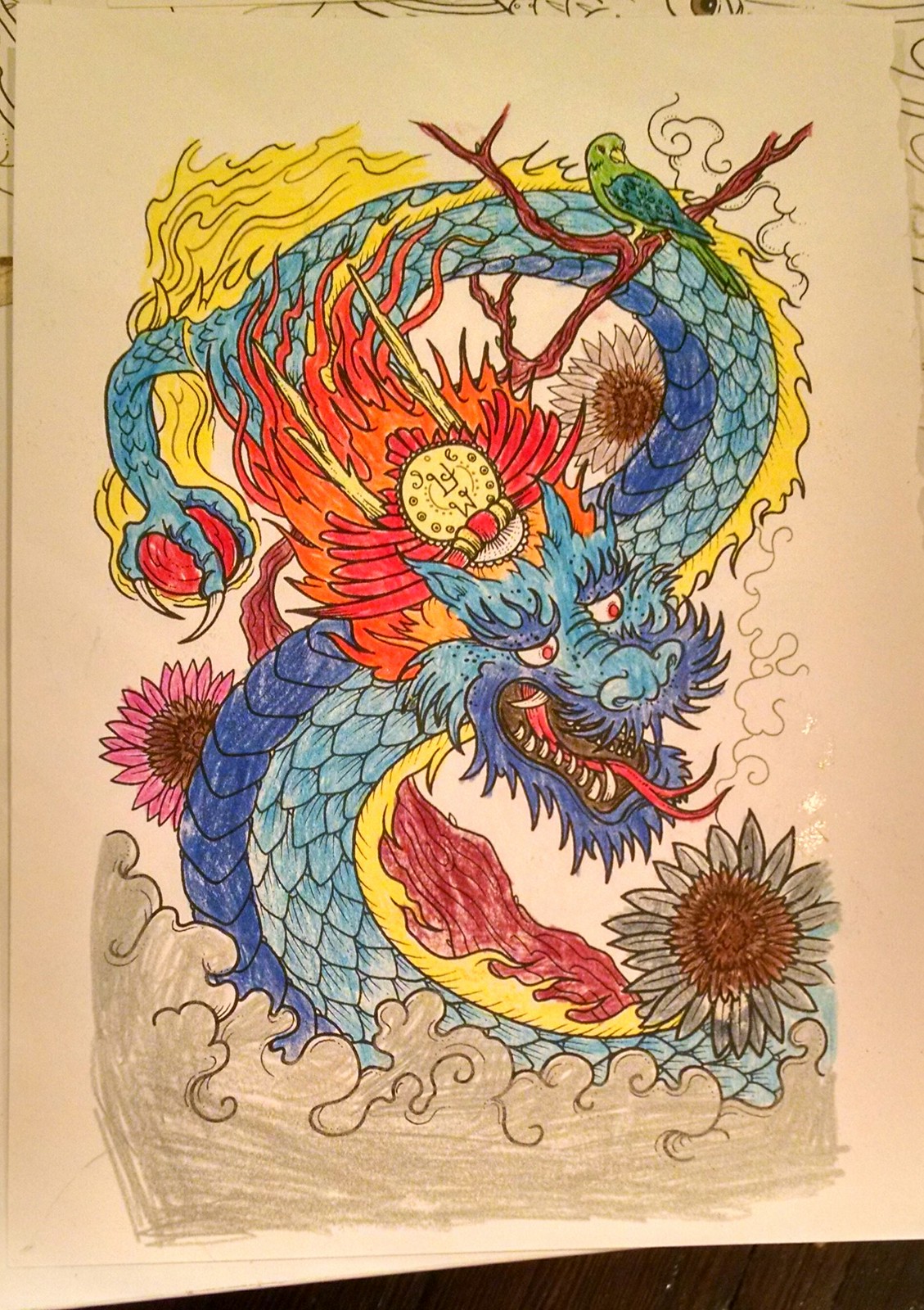The image features a large pink sheet of paper partially overlaying a brown wooden table. On the paper, an intricately drawn dragon is depicted with a combination of light blue and dark blue scales. At the dragon's top, a branch extends outwards, hosting a bird with distinctive plumage—a light green head, a darker greenish-blue wing, and a light green tail. Surrounding the dragon is a manifestation of fiery elements, illustrated in vibrant yellow tones. Clutched in one of the dragon's claws is a bold red ball, adding a vivid focal point to the composition. A delicate pink flower is subtly visible on the side, enhancing the scene with a touch of floral beauty. Beneath the dragon, faint pencil-drawn waves suggest movement or perhaps a watery background. Behind the dragon's head, a large, yellow circular object featuring a dial-like pattern and a red crosspiece adds an element of abstract design. The dragon also sports a forked red tongue and flowing red hair that trails backward. The artwork combines various hues and intricate details, creating a dynamic and captivating illustration.